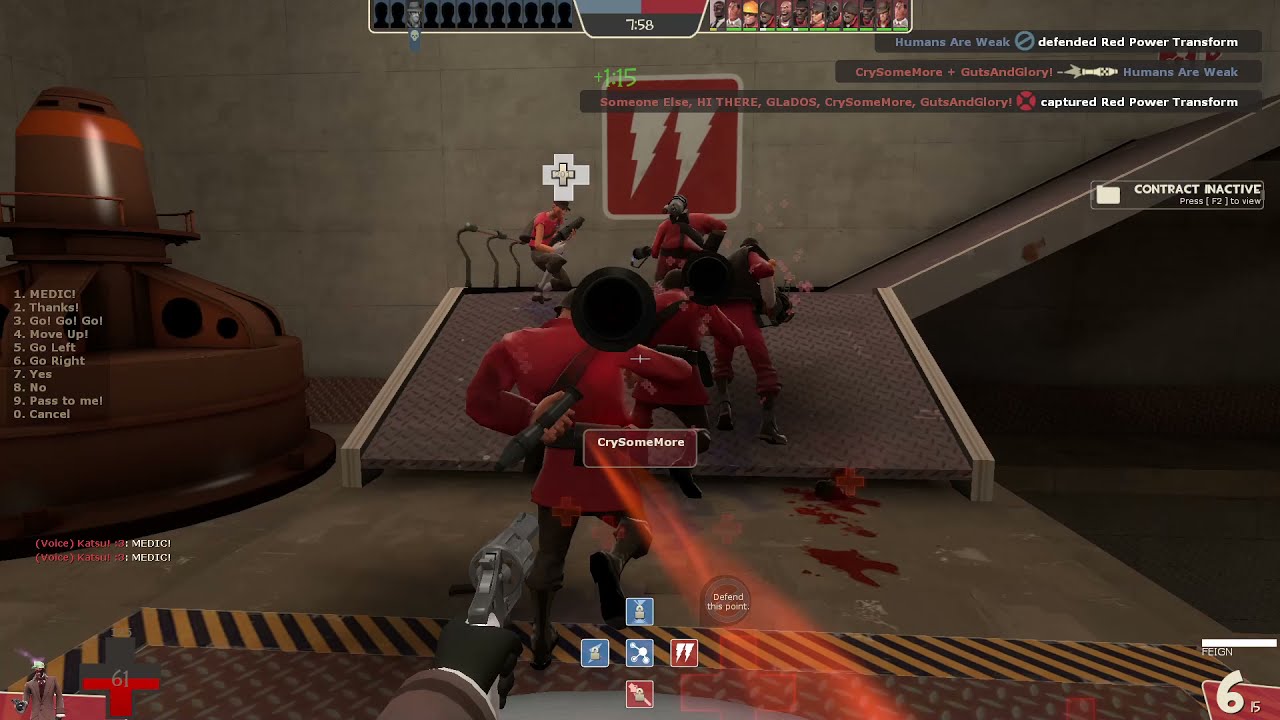The image appears to be a screen capture from a cooperative shooter video game session, taken from a first-person perspective. In this dark, industrial environment with a concrete floor and steel ramp, multiple characters in various shades of red are in action. Some are dressed in uniforms while others sport t-shirts. Armed with powerful weaponry, several characters carry bazookas over their shoulders, one wields a flamethrower, and others grip various lethal instruments. The player, donning a black glove, holds a silver revolver as they progress up the ramp alongside the team. In front of the player is a user named CrySomeMore, indicated by a sign above the character. This character also has a red laser emanating from a device in their hand, appearing to lead the charge across a black and yellow caution line on the floor. The surrounding scene is filled with shades of brown and gray, indicative of an industrial setting, with a concrete wall adorned with a prominent red sign featuring white lightning bolt symbols. Above the action, game interface elements display objectives such as "Defended Red Power Transform," "Captured Red Power Transform," and "Contact Inactive," alongside other vital gameplay information.